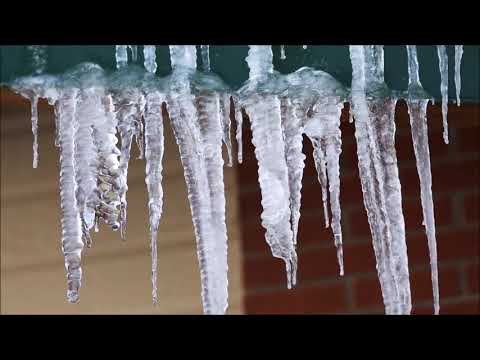This close-up shot captures a cluster of at least 20 icicles hanging from a green structure, which appears to be a gutter or possibly a steel girder beam. The icicles, formed over time, exhibit textured ridges and taper from thicker tops to sharp, pointed ends. They glisten in the light, showing no signs of melting or dripping. In the background, the upper and lower edges of the image are bordered by black horizontal stripes, reminiscent of widescreen bars. The backdrop features a two-part wall: the left half is clad in beige siding while the right half displays faintly lined red bricks. The icicles dominate the image, creating a stark contrast with the varied textures and colors of the background surfaces.